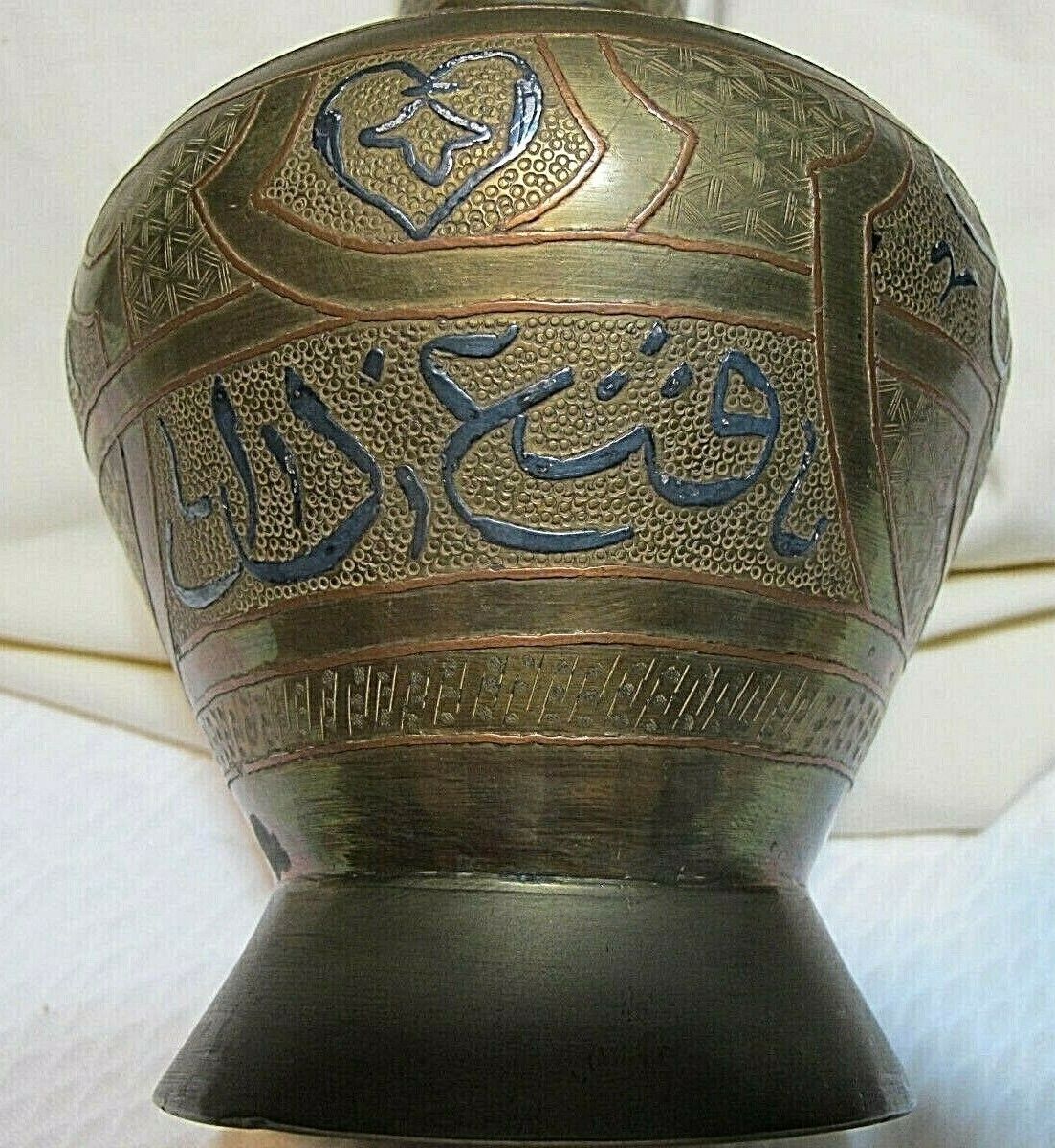The image shows an ancient artifact that resembles a jar or vase with a unique design. It features a flat hexagonal base that transitions into a three-dimensional, vase-like structure. The primary color is a metallic gray with a mix of bronze and gold accents. The body of the vase is decorated with detailed inscriptions and calligraphy-style writing in a dark pewter or navy color, which seem to be in a foreign alphabet. Central to the design is a distinctive blue heart-shaped emblem with intricate details inside, possibly including a diamond or airplane-like shape. Intricate patterns, hammer marks, and vertical lines wrap around the vase, adding to its ornate appearance. The artifact is displayed against a white and cream background, possibly resting on cloth, giving it an antique and cultural essence.